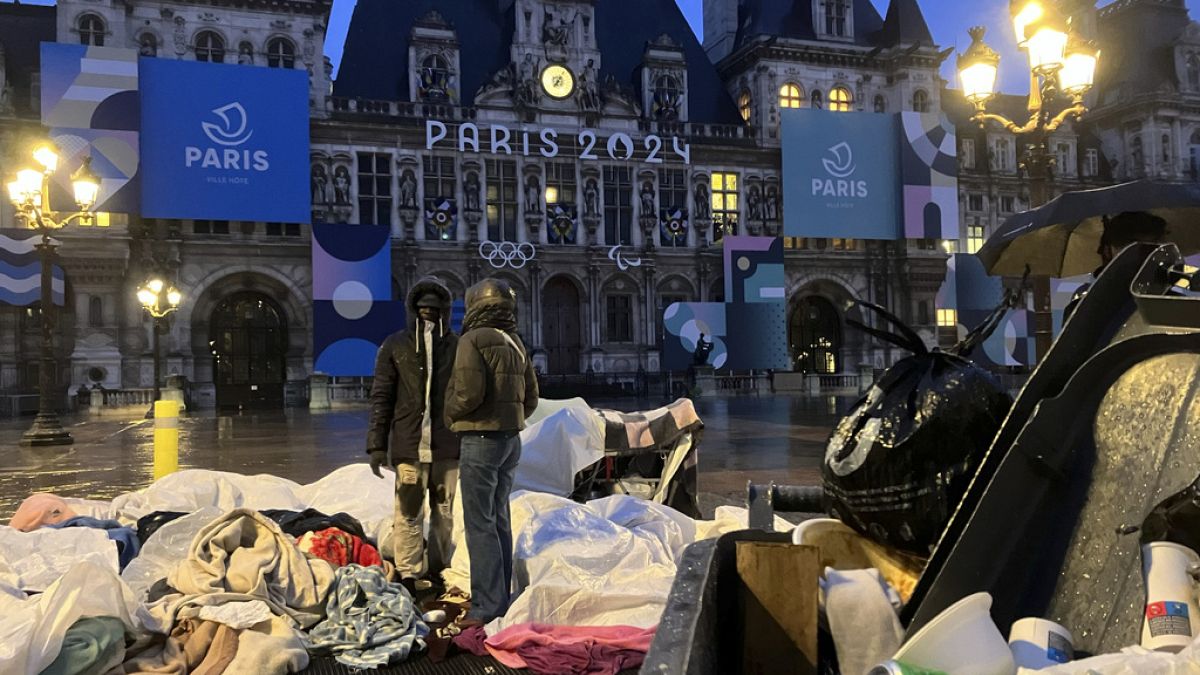This detailed landscape photograph features a grand, castle-like building in Paris, adorned with prominent signs reading "Paris 2024" and displaying the Olympic Rings. The building, built of stone with many arches and numerous windows, transitions from a beige color at the top to a grayer hue at the bottom. An illuminated clock with an unreadable face sits above these signs, casting a soft glow. The courtyard in front of the building is strewn with various piles that resemble blankets or clothes, suggesting a somewhat chaotic scene that might initially be mistaken for a crime scene or a clutter of trash. Scattered among the clothes are plastic bottles, cups, paper, and other miscellaneous garbage items, as well as a sealed black bag within a nearby dumpster. Two individuals stand amidst the debris; one wears a black jacket with a hood, black beanie, beige pants, and black gloves, while the other dons an olive gray hoodie and similar outerwear with jeans.

The wet and reflective sidewalk indicates recent rain. Traditional street lamps with multiple bright lights line the front and sides of the courtyard, enhancing the eerie atmosphere. Banner-like square flags with the Paris 2024 logo and 'Paris' written in large white letters hang on the building's surface. Some windows are lit, suggesting that the building is occupied. The overall scene is one of preparations for the upcoming Paris 2024 Olympics, set against a backdrop of clutter and dampness typical of a bustling urban environment.